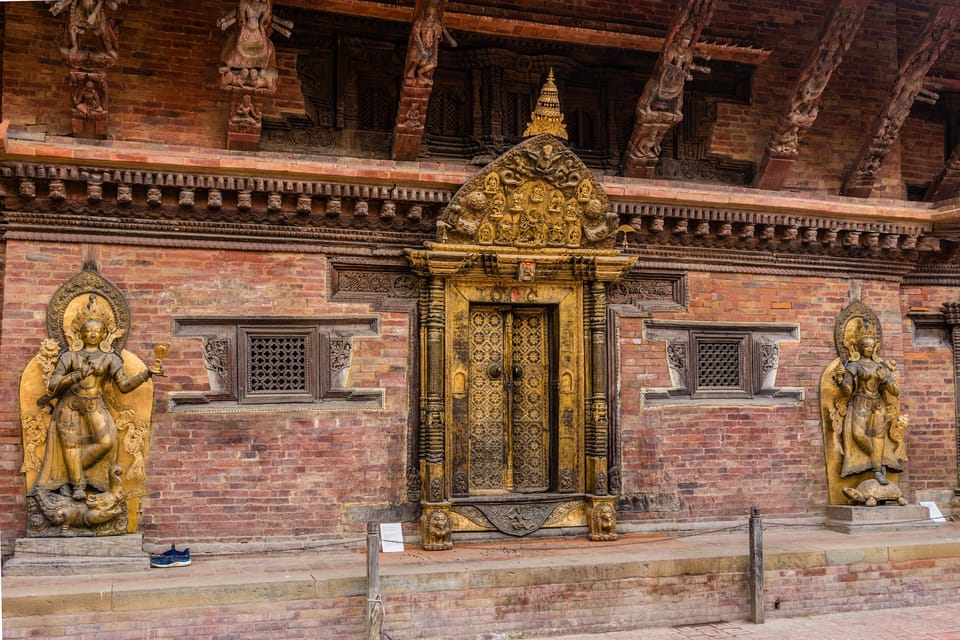The image depicts the ornate facade of a religious building, reminiscent of an ancient temple. The lower part of the structure is constructed from bricks, grounding the majestic gold-plated double doors that serve as the focal point. These doors, adorned with an elaborate black and diamond pattern, are topped by an arch embellished with intricate carvings of various characters and symbols. Flanking the entrance are two identical statues of golden bronze, each depicting a woman in a poised stance, with one knee bent and fingers touching in a delicate gesture. The upper portion of the facade features wooden beams intricately carved, supporting the structure's second floor. Above the doorway, more carvings and religious figures adorn the brick background, adding to the temple’s sacred ambiance. The overall color palette consists of reds, oranges, browns, golds, and touches of white, enhancing the timeless and venerable appearance of the building.